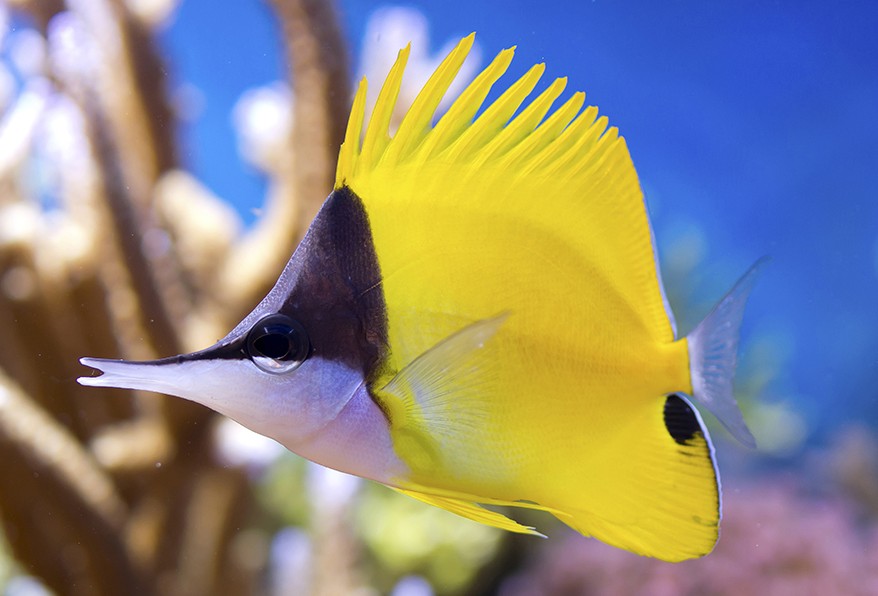This image features a highly unique, possibly computer-generated coral fish, predominantly yellow with distinct markings. The fish's head displays a stark bicolor pattern: the top half is dark gray, while the bottom portion is white, with its eye also split into black and white. Its body, shaped somewhat like an angelfish, is mostly yellow, transitioning into a long, skinny nose. A notable black dot adorns the area near its tail, and its elongated, feather-like fins—also yellow—add to its striking appearance. The backdrop is predominantly blue, indicating an underwater setting, with blurred details of various corals. To the right, there's a subtle mix of pinkish-tan and to the left, stick-like coral formations, culminating in a vibrant depiction of a coral reef ecosystem. This small fish, with its peculiar shape and vivid coloration, stands out as the clear focal point amidst the blurred marine environment.